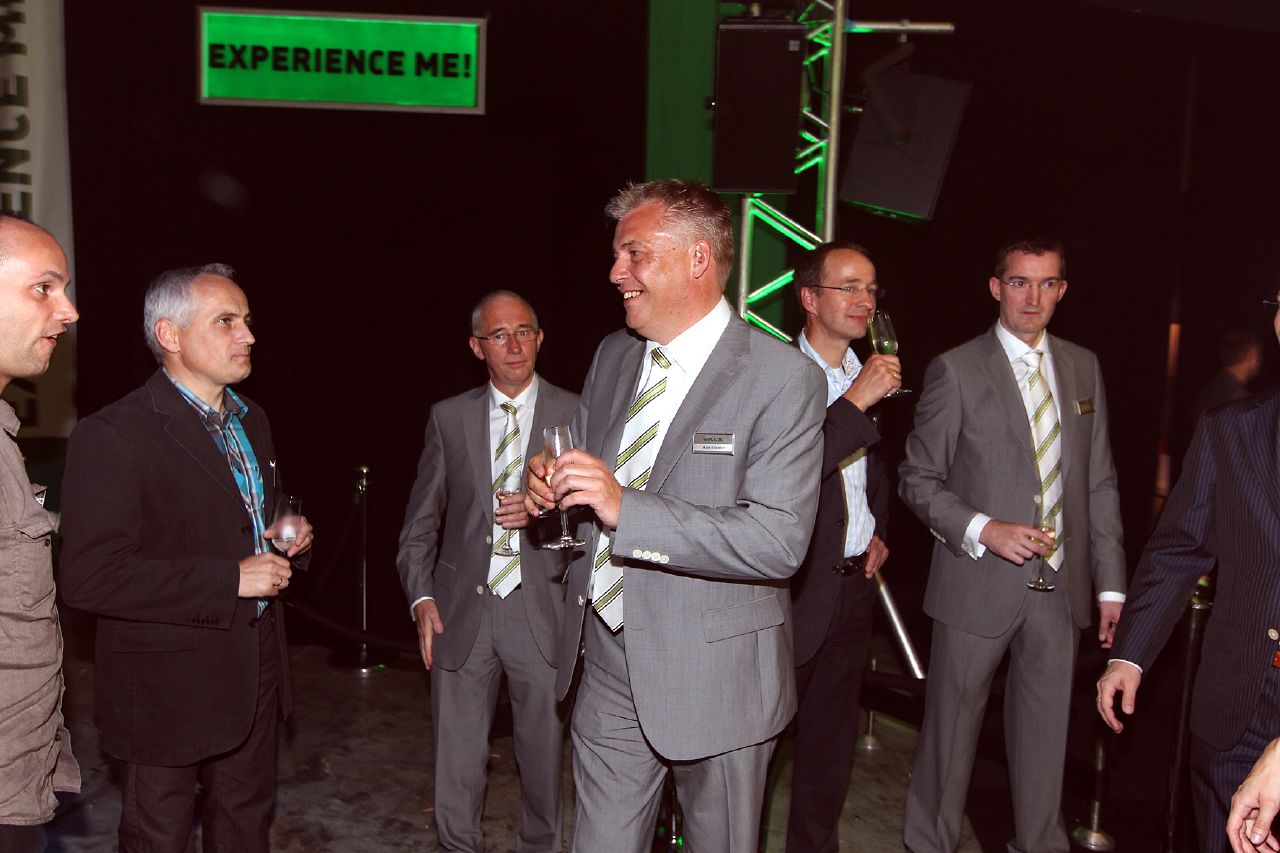The image depicts seven middle-aged men, all dressed in suits and ties, gathered in a somewhat dimly lit room. Each man holds a champagne glass, suggesting they are at a celebratory event or formal gathering. Notably, there is a repetition in their attire—three of the men are wearing identical gray suits paired with white shirts and light green ties. Starting from the left, one man is only partially visible. Next to him stands a man in a brown suit with gray hair. To his right is another man in a gray suit, glasses, and the aforementioned white and light green tie. Beside him is another man in a matching gray suit. To the right of this group is a man in a darker suit with a white shirt. Further right, another man in the same gray suit and tie ensemble wears glasses. Behind them, a green sign with the black text "Experience Me" is visible, along with a staged setup featuring green lighting and silver pillars. Seven men are clearly visible, while an eighth man blends into the darker background on the right side of the picture. The setting appears to be a formal event given the attire and champagne glasses.